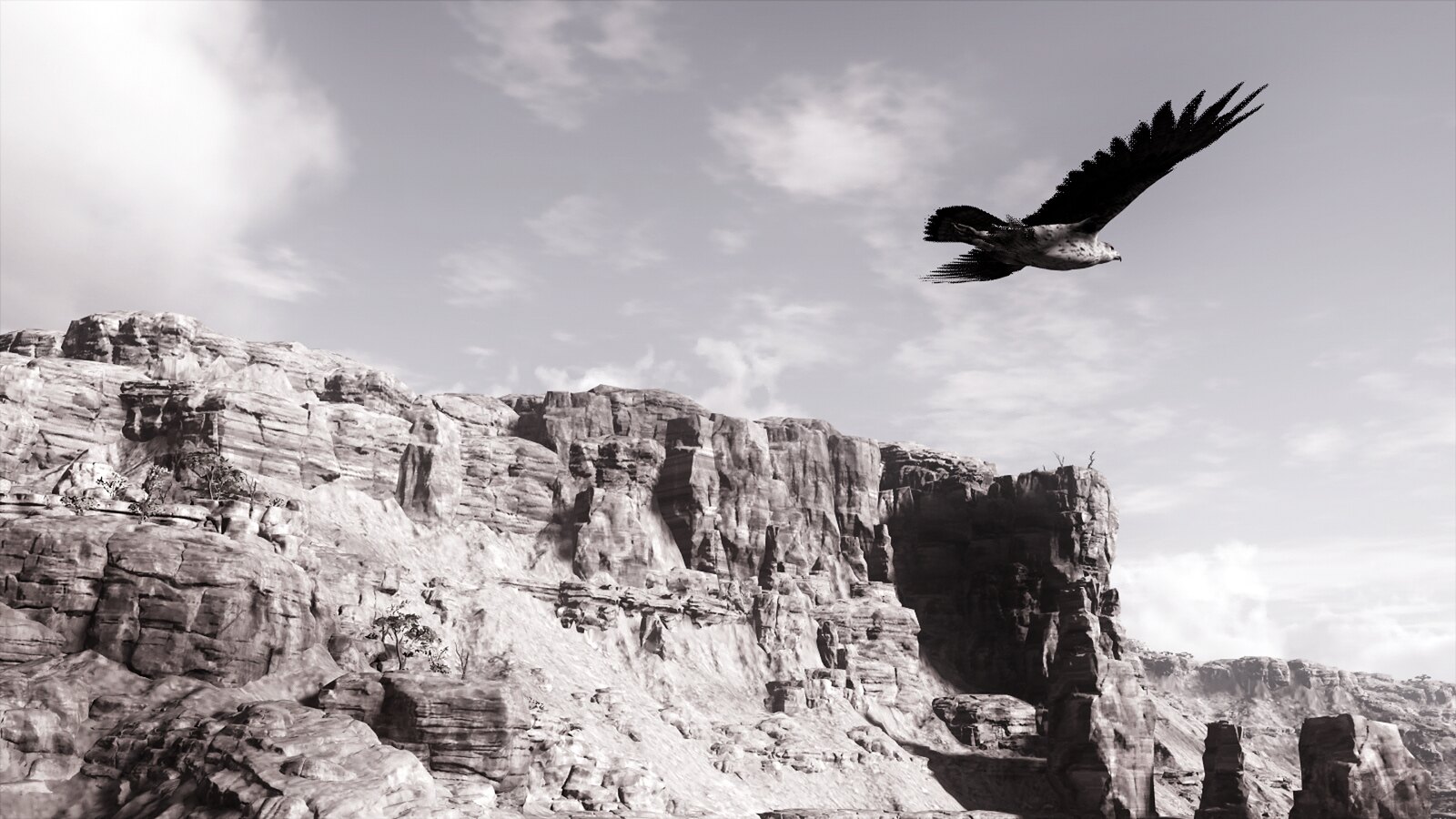This black-and-white photograph captures a majestic eagle soaring through the rugged terrain of a canyon, likely resembling the vastness of the Grand Canyon. The scene is dominated by towering rock cliffs that ascend over half the height of the image, framing the eagle's powerful flight. The eagle, with its wings fully outstretched and tail feathers trailing straight back, glides effortlessly through the gray sky, which is dotted with fluffy white clouds. The bird’s dark wings contrast sharply against its lighter belly, and its pointed beak is distinguishable even from a distance. Positioned about three-quarters to the right of the frame and slightly facing away from us, the eagle commands attention as it navigates the jagged landscape, making for a breathtaking and serene moment frozen in time.